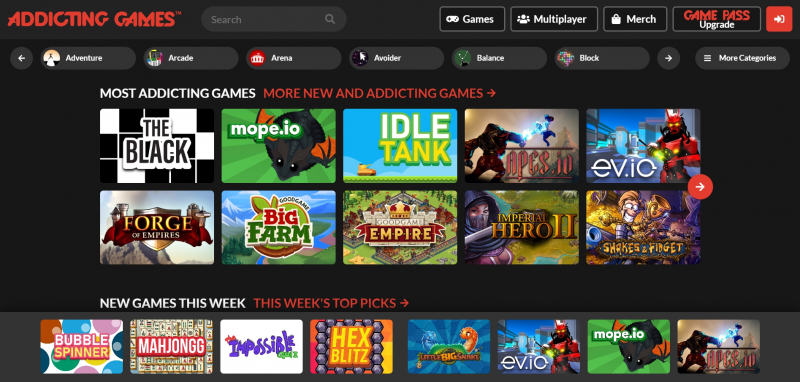This image captures a vibrant screenshot of the Addicting Games website, which features a black background that makes the colorful game thumbnails pop. The website offers various game categories including Adventure, Arcade, Arena, Avoider, Balance, and Block, with more options accessible via a right arrow. In the center lies the "Most Addicting Games" section, showcasing top games like The Black, Mopey.io, Idle Tank, Apes.io, Eevee.io, Forge of Empires, Big Farm, Good Game Empire, Imperial Hero 2, and Shakes and Fidget. The bottom of the page highlights "New Games This Week" and "This Week's Top Picks," featuring titles such as Bubble Spinner, Mahjong, Impossible, Hex Splits, Little Big Snake, Eevee.io, Mopey.io, and Apes.io. Notably, Eevee.io, Mopey.io, and Apes.io appear across multiple categories, emphasizing their popularity.